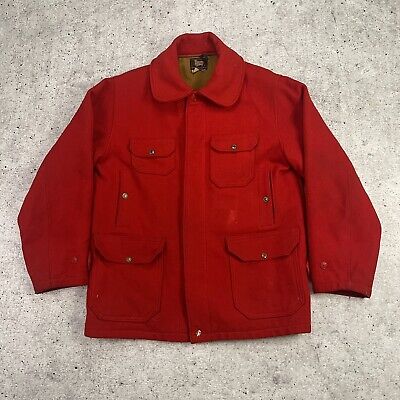The photograph captures a red, long-sleeved jacket laid flat on a light gray, black-speckled concrete surface, suggesting it’s being displayed for potential sale. The jacket features a turned-down collar and appears to be fastened with a zipper, discreetly concealed, accompanied by gold-colored buttons visible at the top and bottom. Additionally, the jacket incorporates a combination of six pockets: two smaller breast pockets on the chest, two hand-warmer pockets with side slits, and two larger pockets at the hip area. The fabric shows signs of wear, suggesting it's not brand new. The sleeves are notably thick, casting heavy, dark shadows. The interior appears insulated, likely brown lining, indicating it’s designed for warmth. A black tag with white writing is noticeable at the neckline, though the specific details on the tag are not discernible due to the image quality. A white stand partially visible on the right side hints at an organized display setup.